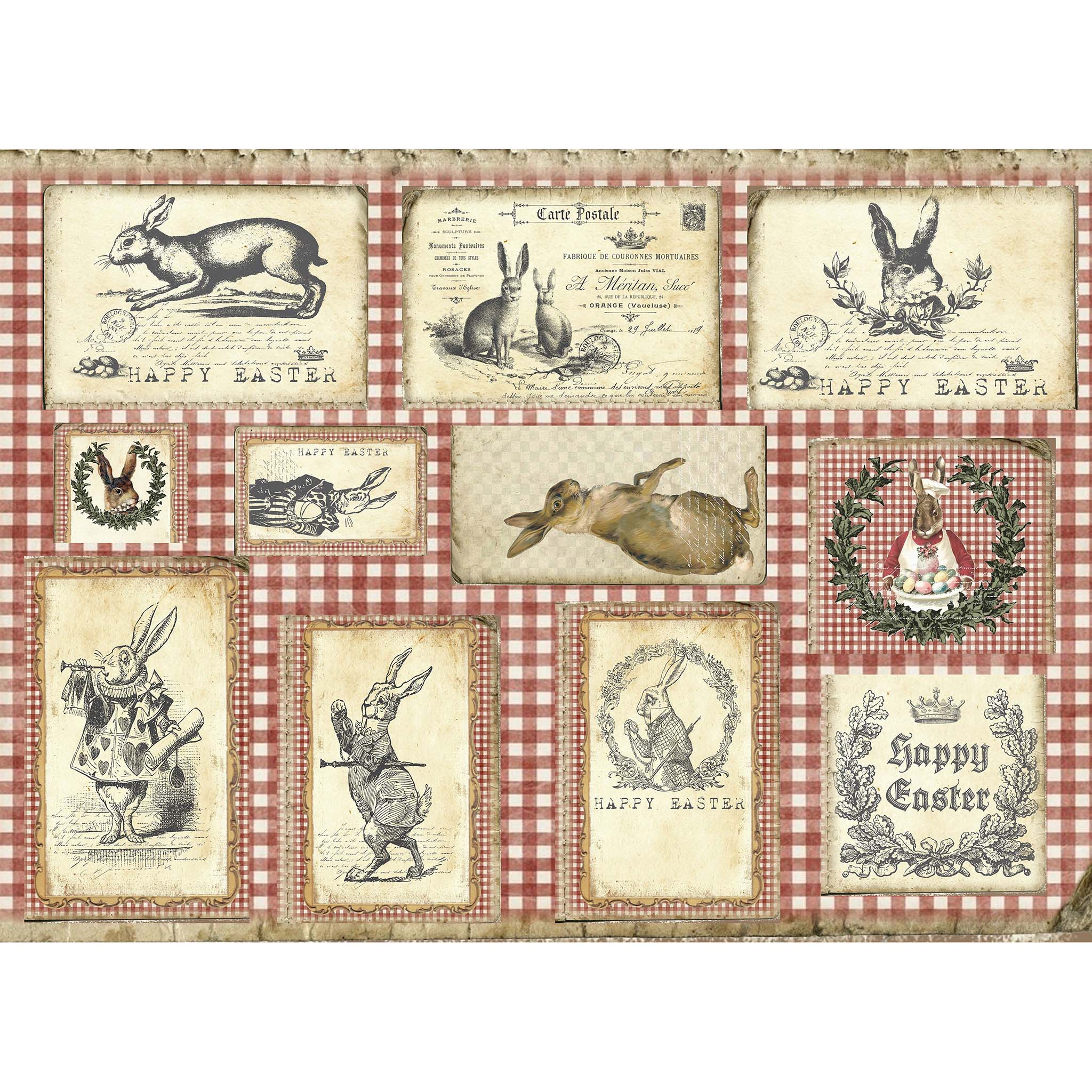This picture showcases an intricately detailed hanging quilt or tapestry adorned with multiple Easter-themed illustrations, primarily featuring bunny rabbits. There are eleven distinct patches, bordered by a red and white checkered gingham pattern. The majority of the patches are vintage, sketch-like images in black and white with a beige or yellow off-white background, while a few sport colored details. Five of the patches prominently display the phrase "Happy Easter." Notable designs include a rabbit in a white and red shirt sitting in front of multi-colored eggs with a green wreath around it, and another rabbit standing upright, walking with a cane. The lower right patch features "Happy Easter" with flowers, leaves, and a small crown above it. The centrally located patch is colored, depicting a brown-furred rabbit. Additionally, the quilt features recognizable characters such as the rabbits from Alice in Wonderland and Peter Rabbit, along with various illustrations reminiscent of old books and vintage advertisements.